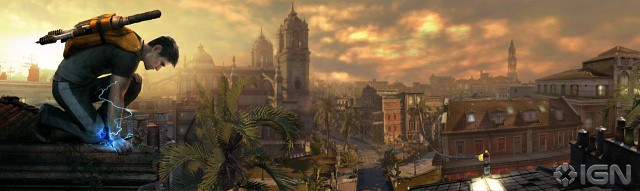In this panoramic screenshot from a video game, the left side of the image features a character kneeling with one knee on the ground while their other knee is propped up. The character supports themselves with an outstretched arm as they look either over the ledge of the building or down at the ground. They have short hair and fair skin, wearing a t-shirt and pants with a distinctive white stripe along the sides. A yellow backpack filled with objects, possibly weapons, is slung over their back.

The character is positioned high on a structure, and the right side of the image reveals a cityscape of an old foreign city that resembles either an ancient English or Arabic town. The city features various-sized buildings, some resembling cathedrals or towers. The skyline is shrouded in a stormy sky with a mix of oranges and grays, suggesting a possible sunset. Scattered among the cityscape are palm trees, adding to the exotic ambiance.

In the bottom right corner of this banner-like, wide-format image, the IGN logo along with the IGN symbol is visible, identifying the source of the screenshot. The overall scene is atmospheric and dramatic, showcasing a blend of architectural styles under a moody sky.